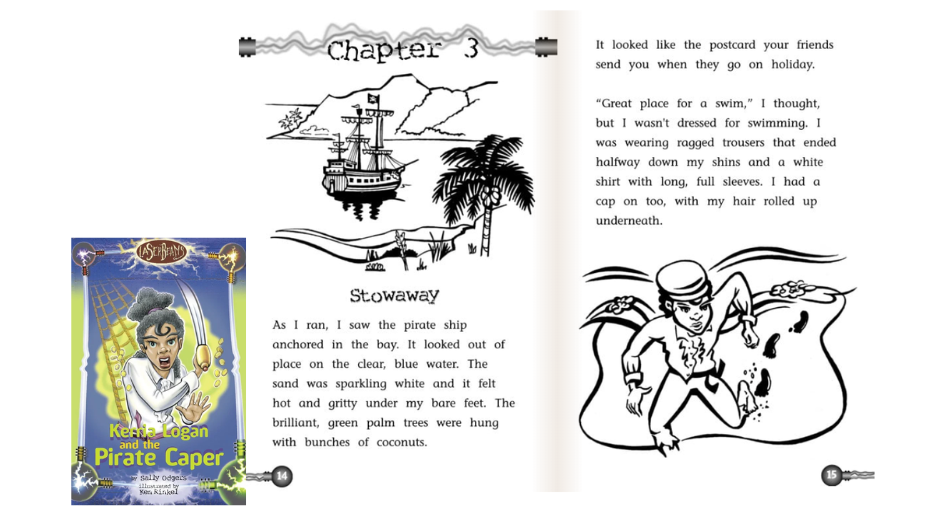The image is a detailed snapshot from the storybook "Kenna Logan and the Pirate Caper" by Sally Rogers, illustrated by Clara Rehn-Griffith. The background of the image is white, with the cover page of the book prominently displayed in the left-hand bottom corner. The cover shows a young woman of African descent with gray-colored, curly long hair, looking frightened with her mouth open. She is wearing a white shirt and holding a sword with a gold handle, set against a background of a net, green designs, and flying gold coins. The title, "Kenna Logan and the Pirate Caper," is in green and blue colors.

The central image, framed by bulbs connected by wires, shows a sketch in black and white depicting a tropical scene. The scene includes a pirate ship anchored in clear blue water, mountains in the background, and an island with brilliant green palm trees laden with coconuts and sparkling white sand. The heading at the top reads "Chapter 3 - Stowaway" with the page numbers 14 and 15 referenced.

The accompanying text describes a character, likely Kenna, dressed in ragged trousers ending halfway down the shins, a white shirt with long full sleeves, and a cap with hair rolled underneath. She is depicted running barefoot on the hot, gritty sand, feeling out of place among the picturesque scenery that resembles a holiday postcard. The text also portrays her thoughts, noting that it would be a great place for a swim, though she isn't dressed for it.

In summary, the image captures the adventurous and vivid setting of Chapter 3, "Stowaway," from the "Kenna Logan and the Pirate Caper," blending the elements of a classic pirate tale with the natural beauty of a tropical island.